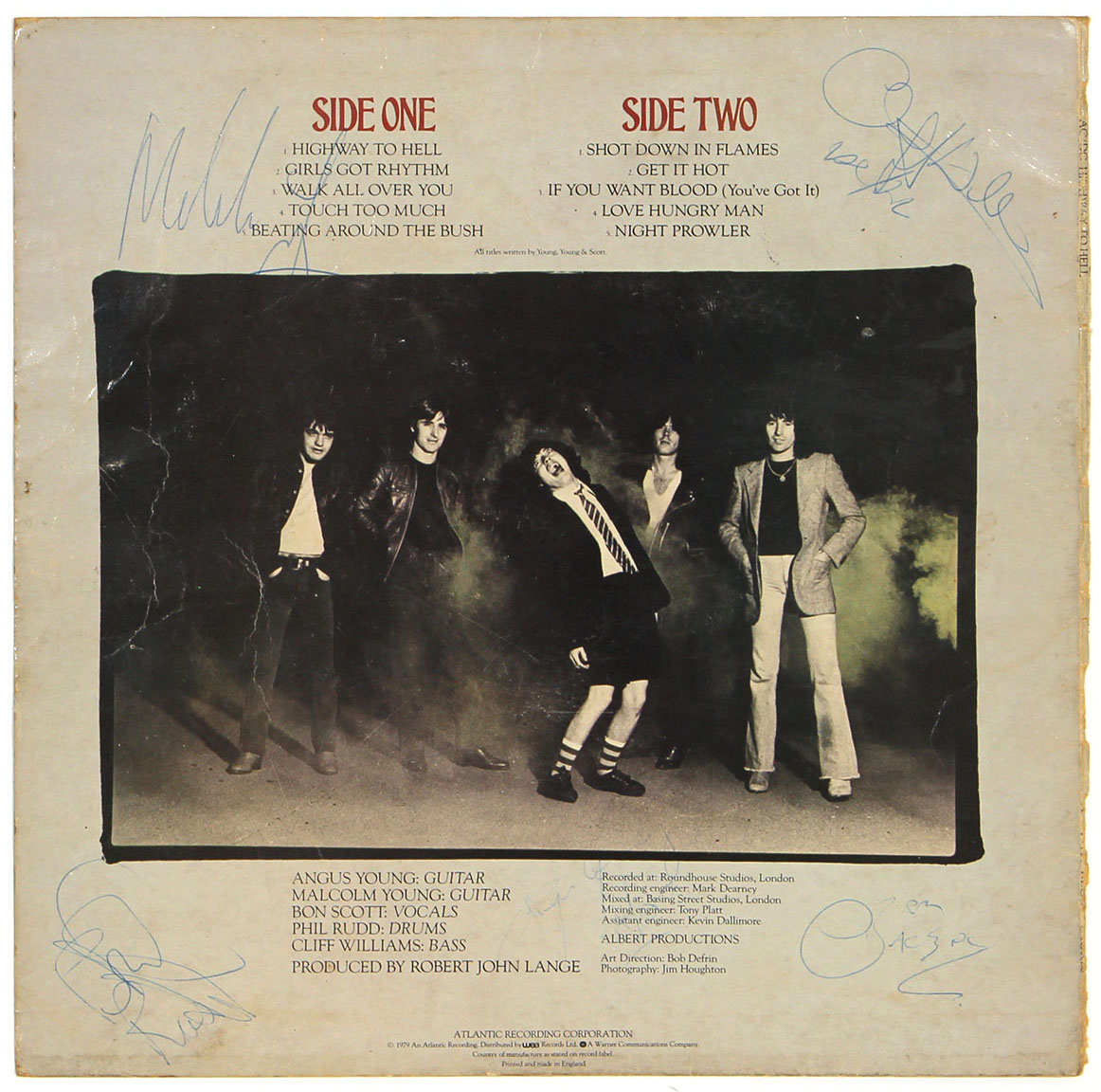This appears to be the back cover of an ACDC vinyl record jacket, showcasing the wear and tear indicative of being an original pressing from the 70s or 80s. It features a weathered, white paper cover with a prominent black-and-white photograph of five young men, presumably the band members, with the central figure in a schoolboy suit, complete with black shorts and a striped tie, striking a dynamic pose. Surrounding the photograph are four blue scribbled signatures, adding a personal touch to the cover.

At the top, the text "Side 1" and "Side 2" is highlighted in red, with the track listings in black text. The Side 1 songs include "Highway to Hell," "Girls Got Rhythm," "Walk All Over You," "Catch Too Much," and "Beating Around the Bush." Side 2 features "Shot Down in Flames," "Get It Hot," "If You Want Blood You've Got It," "Love Hungry Man," and "Night Prowler." The listing of musicians and their instruments can be found below the photograph, while additional details about the record company are printed in small text on the left and right sides. This detailed, nostalgic depiction underscores the album's historical and collector's significance, likely confirming it as an ACDC classic.